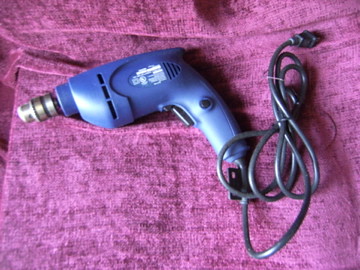The image features a blue electric drill, designed for domestic use or small home repairs, prominently displayed on a purple or maroon-colored blanket, suggesting it is being prepared for sale on an online marketplace like eBay or Amazon. The drill, which has a sleek and smooth appearance, is corded with a black power cable. The cable is either zip-tied or twisty-tied, extending to the right of the drill. The drill lacks a drill bit, and there’s no visible chuck key attached. Manufacturer information, including the model number and warranty details, is printed on the side of the tool. The drill is positioned with the silver drill bit pointing to the left, while the power cord stretches to the right. Both the trigger and a vent for heat dissipation are also evident on the drill.